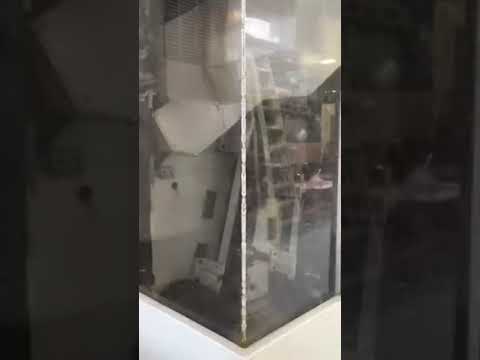The image is a vertical, black and white cell phone photograph focused on the corner of a glass-enclosed structure, resembling a shower-closet or storage area, possibly under construction. The foreground features transparent glass walls, revealing various construction equipment inside, including a collapsible ladder prominently positioned near the center. To the left of the ladder, scattered drywall materials and white ductwork are visible through the glass. Above, ventwork is discernible in the upper middle portion of the image. The floor inside the structure is littered with various items, hinting at ongoing construction. Sunlight streams through a back wall within the glass enclosure, enhancing reflections on the transparent panels. The image is framed by heavily faded, zoomed-in elements of the primary picture, creating almost black borders on either side, which add a sense of depth and focus to the main subject. The base of the structure is white, and small, black rectangular openings can be seen within the enclosure, contributing to the intricate details of the scene.